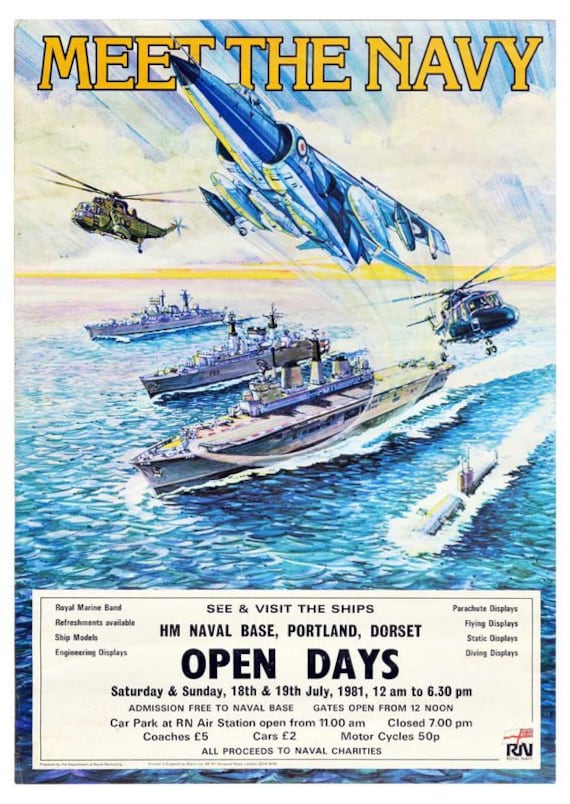This illustrated poster, promoting the "Meet the Navy" event, features captivating imagery and essential event details. Dominating the top of the poster, "MEET THE NAVY" is boldly displayed in large gold capital letters, slightly obscured by a fighter jet flying across the center of the text. Two helicopters flank the jet, positioned a little behind it, contributing to the dynamic aerial scene. Below these aircraft, the ocean sprawls out with four large watercraft: three battleships and a visible submarine near the right side, partially above water.

At the bottom, detailed information about the event is provided. The key announcement reads "See and visit the ships" at HM Naval Base, Portland, Dorset. Highlighted in larger bold text are the dates and times: "Open Days, Saturday and Sunday, 18th and 19th July 1981, 12 a.m. to 6:30 p.m." Additional logistical details include "Admission free to Naval Base. Gates open from 12 noon. Car park at RN Air Station open from 11 a.m., closed 7 p.m. Coaches, £5. Cars, £2. Motorcycles, 50p. All proceeds to Naval charities."

In the upper left corner, smaller text lists attractions such as the Royal Marine Band, refreshments, ship models, and engineering displays. The upper right corner mentions parachute, flying, static, and dive-in displays in similar small text. In the lower right, the initials "RN" appear alongside a small, indistinct red symbol or text. The entire scene and textual details create an engaging and informative invitation to this naval event.